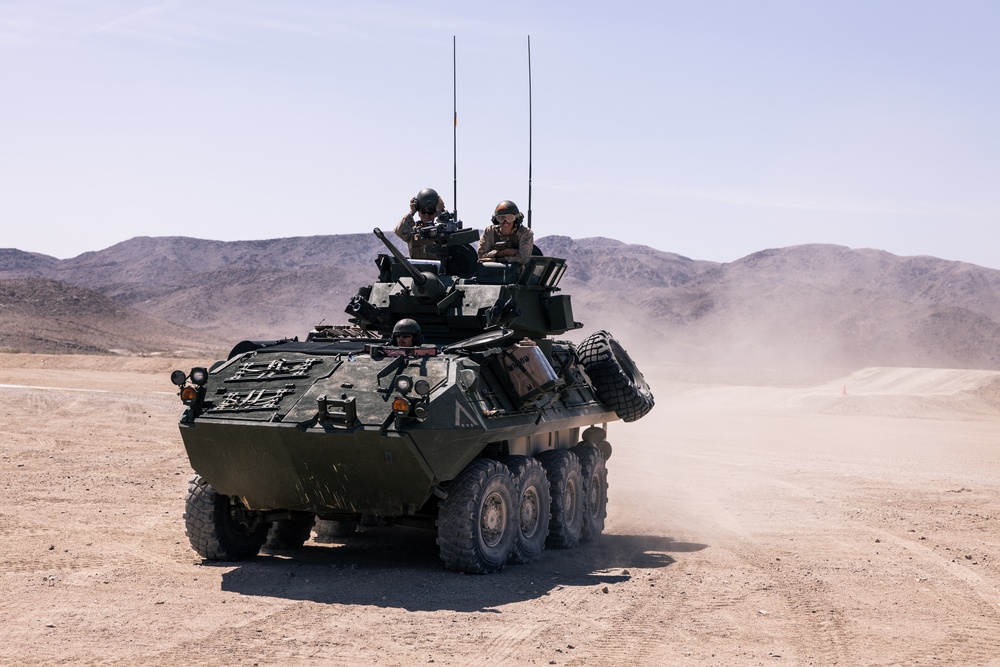In this outdoor image, a green, eight-wheeled military tank is traversing a barren, dusty desert landscape. The sun shines brightly in a mostly clear sky, making for a hot day with only a hint of haze. In the background, a mountain range stretches across the horizon, composed primarily of dirt with barely any greenery. The foreground features a flat, compacted dust area adorned with a few small rocks and marked by the tank's tracks. The tank is positioned towards the front left corner of the image, kicking up clouds of dust as it moves. Three soldiers are visible: two are manning the guns from the upper area of the tank, and one, possibly the driver, has his head poking out from a lower hatch. All are dressed in green uniforms with helmets and goggles. Antennas protrude from the tank, indicating its readiness for communication in the harsh desert environment.